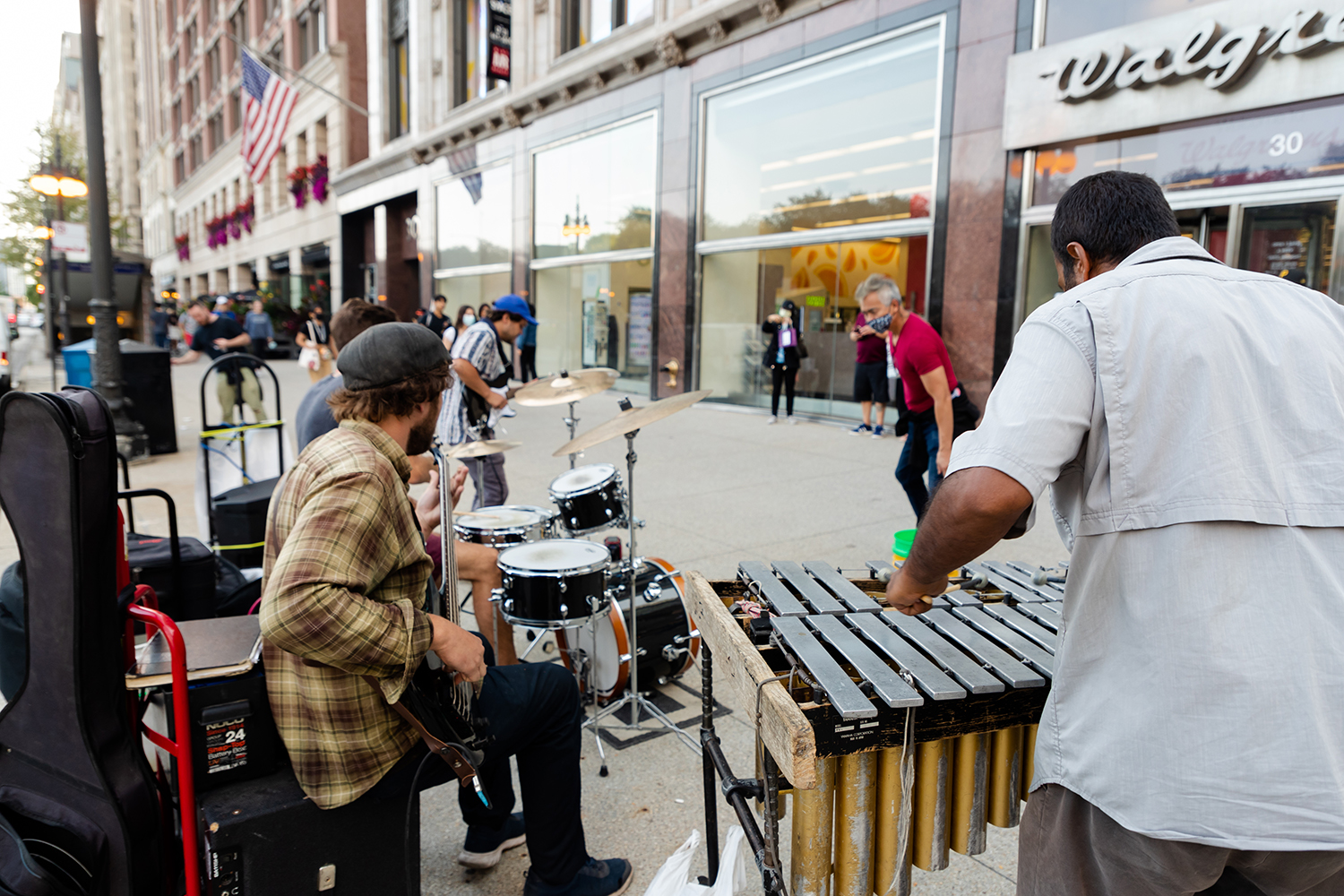On a bustling city sidewalk, likely in New York City, a lively scene unfolds in front of a Walgreens Pharmacy. Tall and massive buildings tower above, framing the street. An outdoor band is set up outside the Walgreens, drawing the attention of passersby. On the right, a slightly overweight man in a white button-up shirt and gray slacks plays a large xylophone, striking its bars rhythmically. His black hair and the back of his head are visible from the viewer's perspective. To the left, a man in a beige checkered shirt, black pants, black tennis shoes, and a gray cotton beret plays an electric bass while seated on a speaker or amplifier. Another man, partially obscured, sits behind a black drum set, his brown hair, legs, and arms visible. In front of the band, a guitarist wearing a white striped t-shirt or button-up shirt and a blue hat plays a black electric guitar. He sports gray pants. A man in a cotton COVID mask, possibly a spectator or a dancer, stands nearby, adding to the dynamic atmosphere. The street is heavily populated, and an American flag hangs from a building window, accentuating the urban American setting. Some people are gathered around, enjoying the music, and perhaps making donations. The vibrant, spontaneous concert captures the essence of city life during the pandemic era.